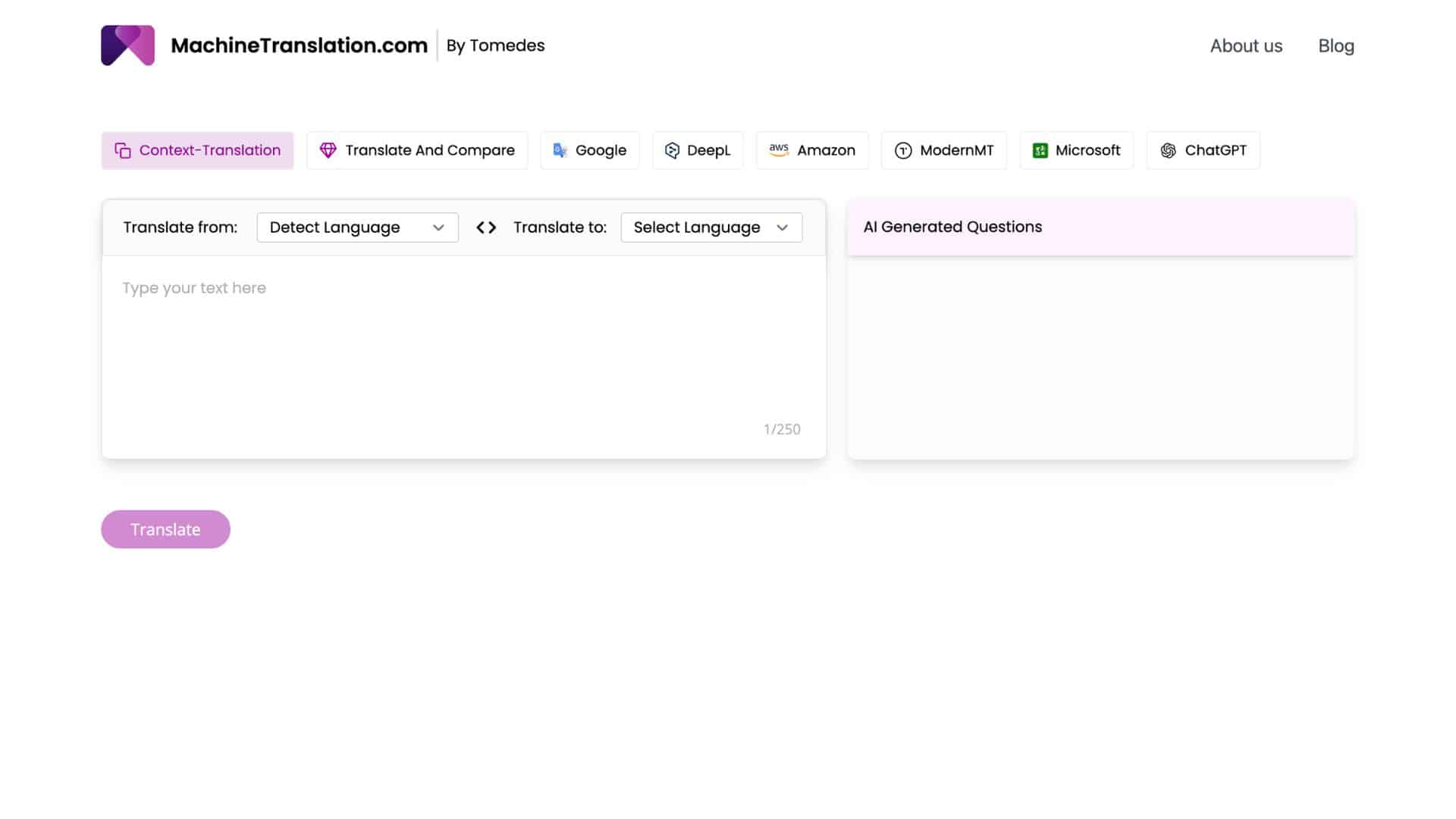This detailed caption describes an image of an online tool interface:

"The photo captures an online translation tool interface displayed against a white background in landscape orientation. In the upper left, there is an icon consisting of a dark purple and light purple intersecting triangle, with a white triangle beneath it, forming a rectangular shape. Adjacent to the icon, the text 'MachineTranslation.com' is written in black font. A thin horizontal or vertical border next to it contains the text 'By Tometes'. To the right, 'About Us' is written in grey font.

Below this header is a highlighted purple box featuring pink text that reads 'Context Translation'. Surrounding it are other options like 'Translate and Compare', 'Google', 'Amazon', 'Modern MT', 'Microsoft', and 'Chat GBT'.

A prominent box spans approximately 60% of the screen width. It contains fields labeled 'Translate From', 'Detect Language', 'Translate To', and 'Select Language'. Within this box is a white text area for inputting the text to be translated, accommodating up to 250 characters as indicated by the notation '1/250' at the bottom right corner.

To the right of this is another box with a pink border and black text that says 'AI Generated Questions'. Beneath this heading is an empty, white, landscape-oriented rectangular box for entering questions. At the bottom of this section, there is a purple 'Translate' button."